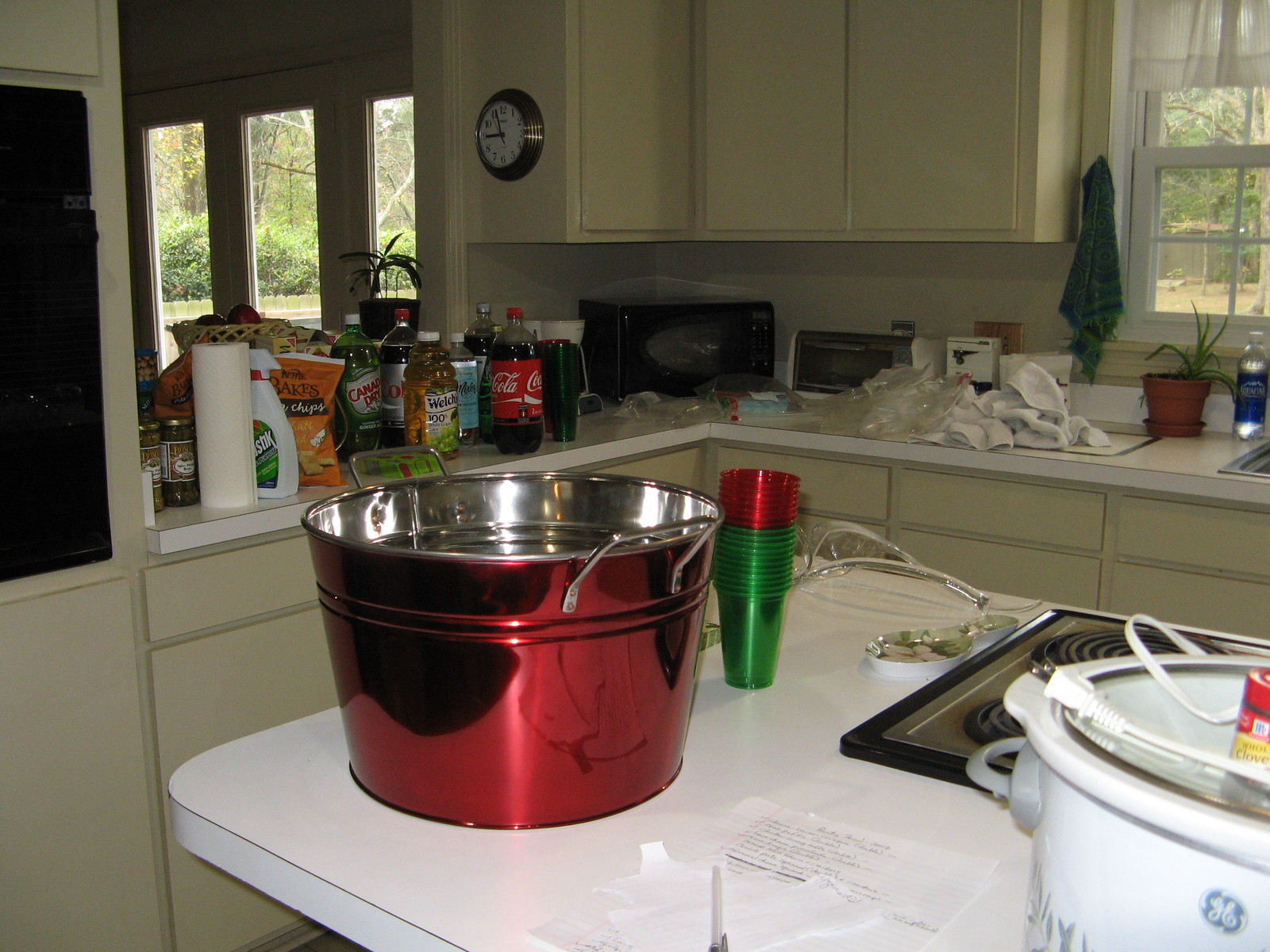Indoor color photograph capturing a detailed view of a kitchen corner. In the foreground, a kitchen island extends diagonally from the lower right corner, covering about two-thirds of the image. The island's white countertop is adorned with various items: 

- A large, round, violet-red container, positioned left of center.
- To its right, a ceramic crock pot bearing the GE logo, with its unplugged cord resting on top.
- Behind the crock pot, there's a stack of approximately 12 green cups topped with another stack of four or five red cups.
- Additionally, a cooking range is partially visible behind the crock pot on the island.

In the background, starting from the left, a portion of the black oven door can be seen. Moving rightwards, the countertop hosts:

- A collection of two-liter soda bottles.
- A roll of paper towels.
- A bottle of cleaner.
- In the corner, a microwave.

Adjacent to the microwave on the right is a white toaster oven, alongside a disordered collection of rags and wrappers. The upper portion of the background features tan cabinets. On the upper right, a window with a curtain reveals a glimpse of an outdoor backyard. Similarly, to the left in the background, patio doors with tall, vertical rectangular windows offer another view outside. Just left of center, mounted on the cabinet wall, a clock indicates the time as five minutes to nine.